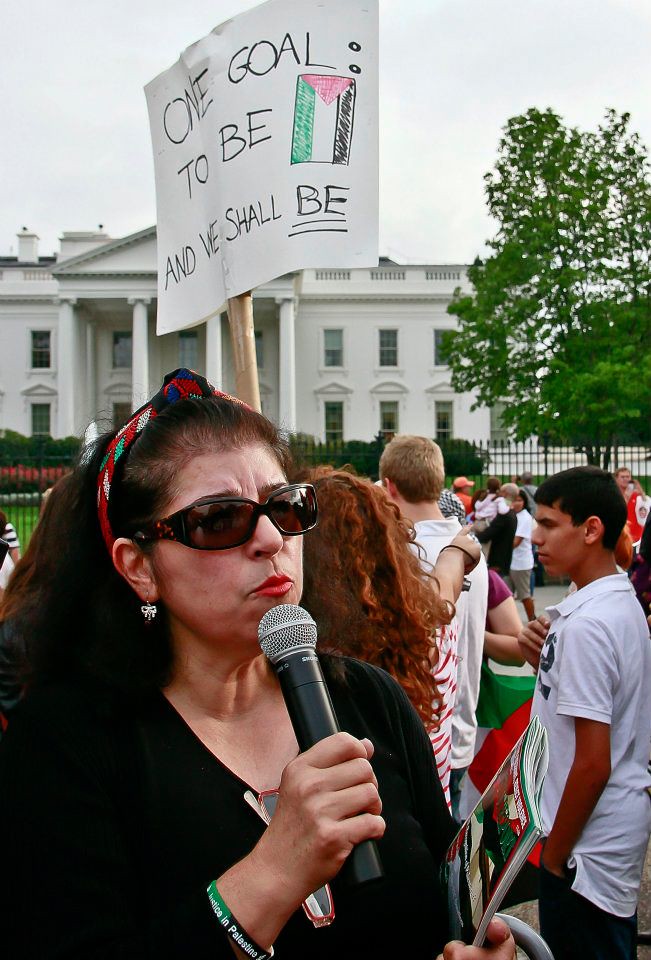In an overcast, pale blue sky day, an outdoor protest is taking place in front of the White House. The scene is dominated by a diverse group of people, including young men and women, gathered behind a metal gate. The focal point is an older woman, possibly in her late 40s, standing in the foreground. She has long, dark reddish hair pulled back with a headband, which features the colors of the Palestinian flag. She wears sunglasses and a black top, accessorized with earrings and a bracelet that reads "Palestine." In one hand, she holds up a microphone to her mouth as if being interviewed, while she clutches a book or magazine in the other. Her lips are pursed, adding a sense of determination to her expression. Directly behind her, a person holds a sign on a stick, prominently displaying the slogan, "One goal, to be, and we shall be," with the second "be" underlined twice. The sign includes an illustration of the Palestinian flag. The backdrop of the scene features green trees and bushes forming a hedge along the fence in front of the iconic White House. The combination of the setting and the elements of the protest suggests a demonstration in support of Palestine.